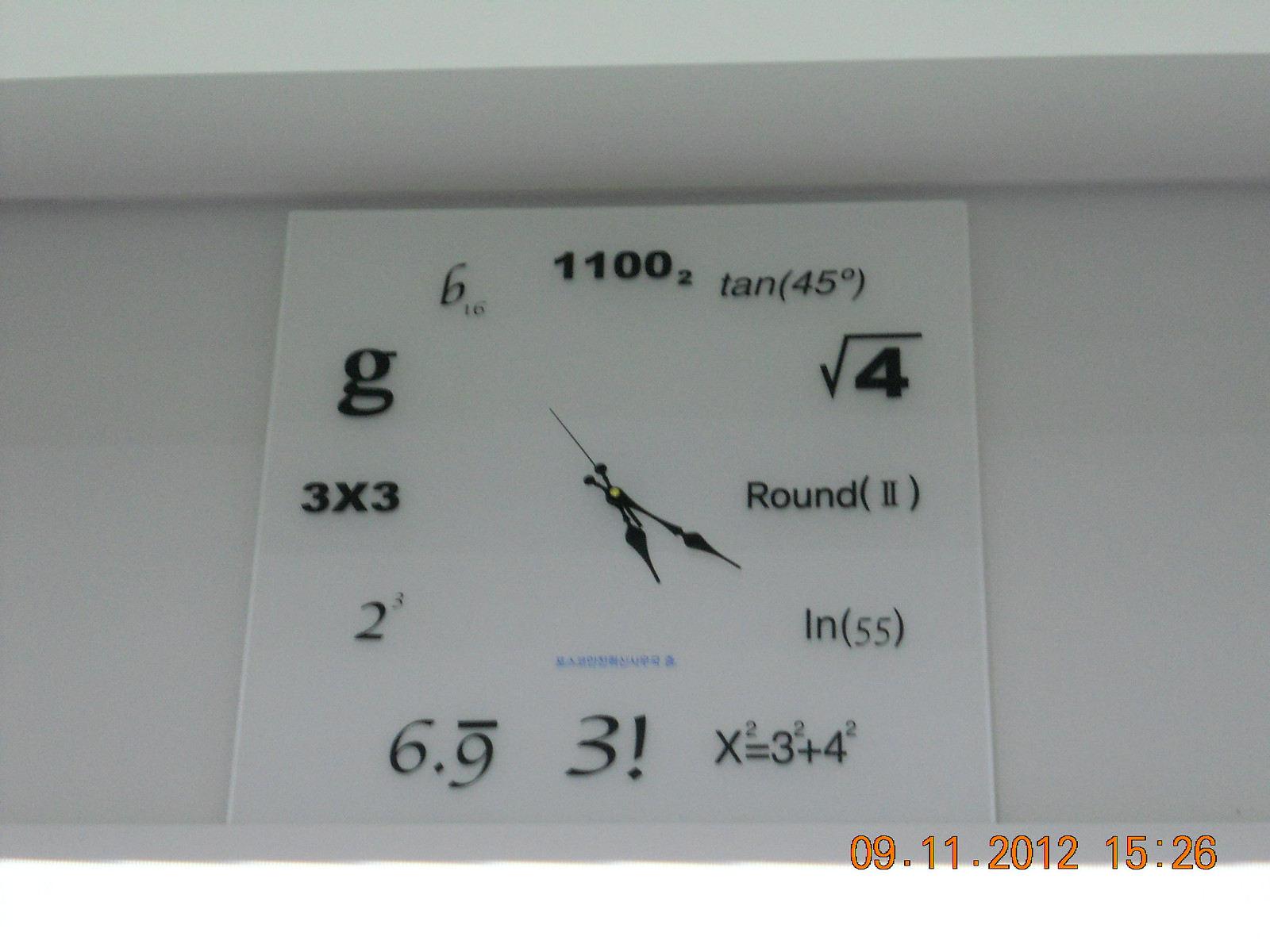A highly sophisticated clock with a mathematical theme, captured on September 11, 2012, at 3:26 PM. The clock features a square design with a white background and black hands and numerals. Surrounding the clock face, various mathematical equations are used to denote each hour. For instance, 11:00 is represented by 11 squared, and 9:00 is indicated by 3 x 3. Among the equations displayed are tan(45 degrees), the square root of 4, and more complex expressions such as x squared equals 3 squared plus 4 squared and 3 factorial. Based on the position of the hands, the time shown is approximately 5:25.